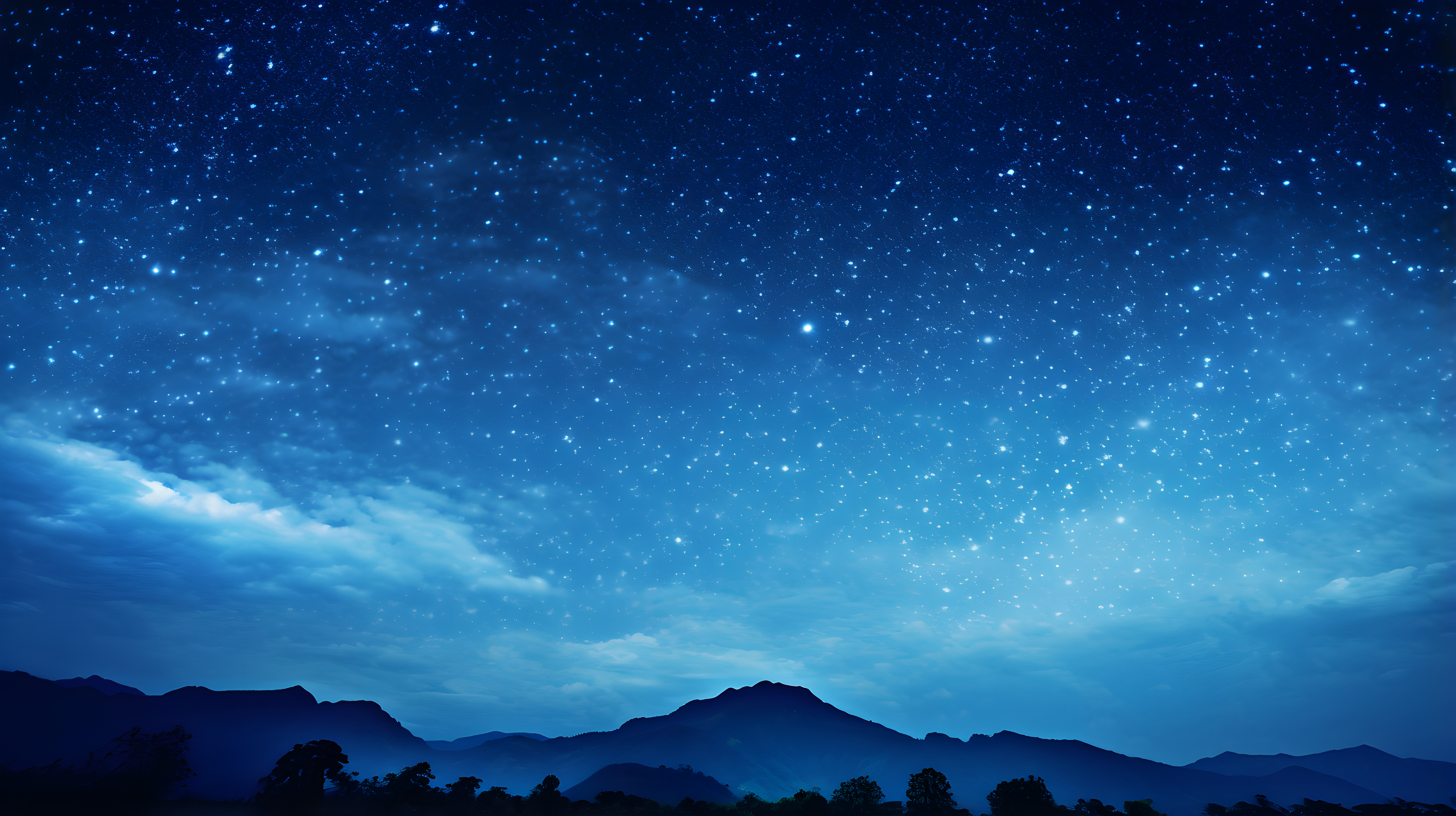The image, which could be a painting, a photograph, or digitally created, captures a serene night sky filled with a myriad of bright white stars of varying sizes. The sky is artistically presented in diverse shades of blue, transitioning from a light blue near the horizon to a deep navy at the top, with scattered, billowing white clouds adding texture. Below the expansive sky, a striking dark blue mountainous range with jagged, pointed peaks rises prominently. Further down, the silhouette of a tree line in rich blackness suggests a dense forest, its forms adding depth and contrast to the scene. The overall composition evokes a tranquil yet awe-inspiring night under a star-studded sky.